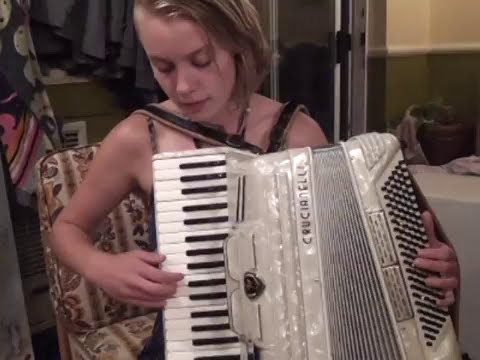In this detailed photograph, a young woman, approximately 18 to 25 years old, is sitting on a beige chair with a subtle floral pattern inside a room that appears to be a rehearsal space. The chair itself has distinct leaf and flower designs in a brown shade. She has blonde hair, which is styled with a swooped section over the right side of her head. She has pale skin and is focused intently on playing a light gray and silver accordion. Her eyes are directed downwards, concentrating on the black and white piano keys of the accordion.

She is holding the accordion with both hands; one hand is poised over the keys, suggesting she is in the middle of playing a piece of music. The accordion is strapped to her, draped across her front, with the piano section clearly visible on the left side of the image. Behind her, the room reveals a blend of a dark green lower wall and a gray upper wall. The setting is somewhat cluttered, with various items strewn about, and an open door can be seen in the background. Additionally, there is an unreadable label running vertically, which partially reads as “Krabuchia” or “Butchia” and another indecipherable label starting with "E-L." The overall scene captures a moment of focused musicality within a lived-in, creatively occupied space.